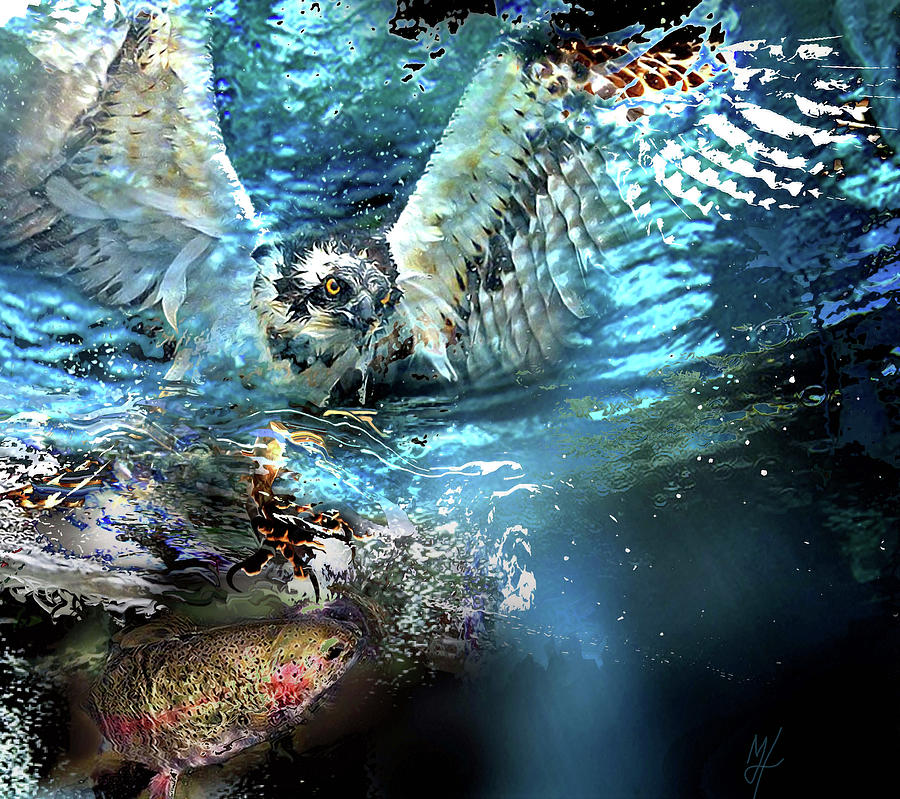This square-shaped painting, executed in either acrylic or oil, presents a vivid and dynamic underwater scene framed under bright sunlight. In the top portion, an owl with striking black and white plumage and yellow eyes is dramatically captured mid-dive, its large wings outspread as it just begins to break the surface of the blue water. The bird's talons are poised to snatch a rainbow trout swimming close to the water's surface, identifiable by its green body and distinctive bright red stripe. Surrounding the owl are splashes and ripples of color, creating a sense of motion and turbulence as the predator disrupts the calm surface. The lower portion of the image, viewed from an underwater perspective, is filled with additional marine life, including various brightly colored fish, a shrimp, and a crab, adding to the painting's vibrant and busy atmosphere. The overall color scheme is dominated by the deep blues of the water and the contrasting white of the owl’s feathers, becoming darker towards the bottom of the painting. An autograph, marked with the initials MJ or ML, is visible at the bottom, adding a personal touch from the artist.